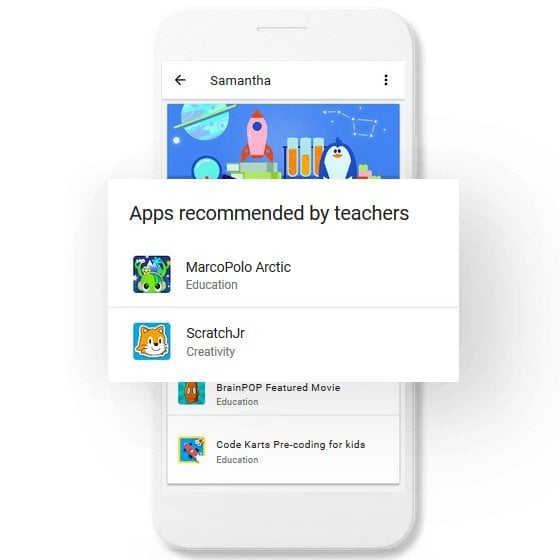Mock-up of a Smartphone Interface:

The image depicts a mock-up of a dark gray smartphone with rounded corners. At the top, there is a white search bar featuring a black arrow on the left, the word "Samantha" in bold black letters at the center, and three ellipses on the right. 

Below the search bar is an intricate image showcasing a planet. The planet is predominantly cyan blue with dark blue splotches on the left and small circles of dark blue mixed with lighter blue splotches on the right side. Surrounding the planet is a glowing white circle. The background features a dark blue sky with the Big Dipper constellation visible on the right side.

In the foreground of the image, a pink rocket ship with red fins and a red top is illustrated, having a small dark blue circular window. It sits atop a teal book and a forest green book. To the left of the rocket ship, a cyan circle with a dark blue border can be seen. To the right, several cylindrical vials are placed on a stand. Further right is a blue penguin with a white belly, orange beak, black eyes, and a tufty dark blue cowlick. Next to the penguin, there are some green plants.

Below this image, a white rectangular pop-up displays a section titled "Apps Recommended by Teachers" in bold text. The section features four app icons with their descriptions:

1. **Marco Polo Arctic**:
    - Icon: A green alien creature with yellow and cyan blue antennae, against a white cloud background.
    - Description: "Education" in gray text below the icon.

2. **Scratch Jr.**:
    - Icon: An orange cat with a white face, black nose, black eyes, and black ear tips.
    - Description: "Creativity" in gray text below the icon.

3. **BrainPOP Featured Movie**:
    - Icon: An orange fish-like character with white eyes.
    - Description: "Education" in gray text below the icon. The text "BrainPOP" has the 'B' and 'P' capitalized.

4. **Kode Karts: Pre-Coding for Kids**:
    - Icon: A red car with black wheels emitting white smoke, set on a yellow-bordered blue background.
    - Description: "Education" in dark gray text below the icon.